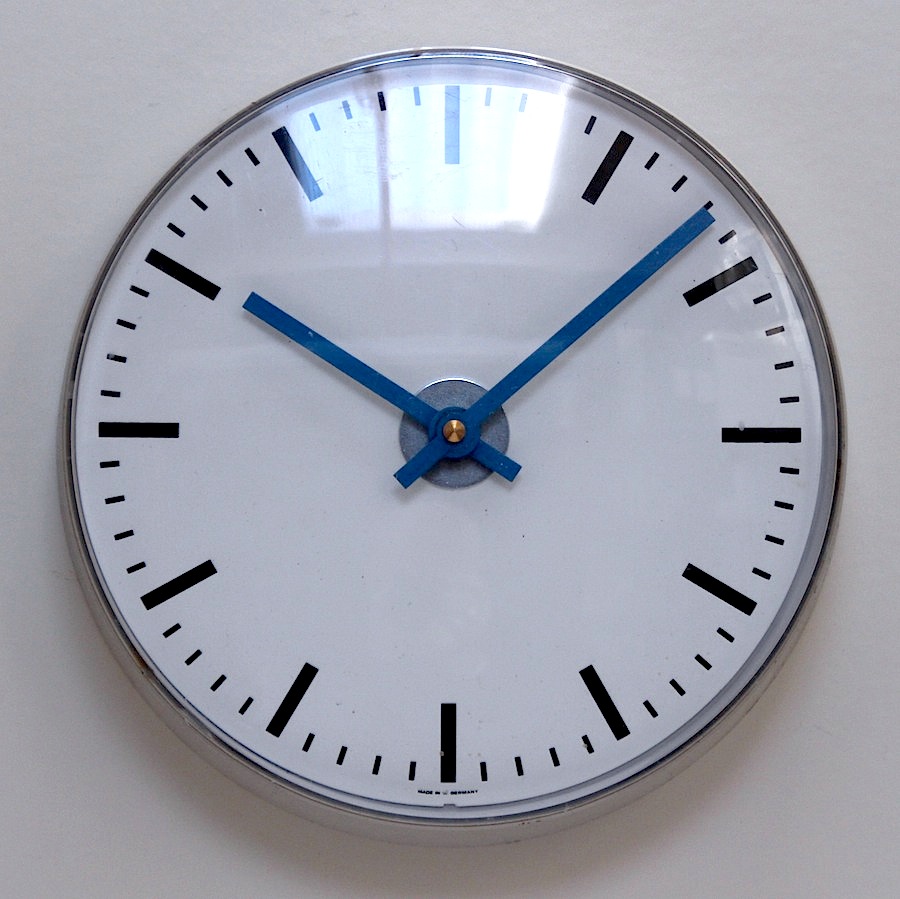The close-up photograph captures a minimalist wall clock set against a lilac-gray wall. The clock features a sleek circular design with a silver-toned metal rim. A soft reflection, likely from a nearby window, casts a bright square and a smaller rectangular shape onto the clock's surface, adding a touch of dimension. The clock's face is devoid of numbers; instead, it displays twelve thick, solid lines at the hour marks, complemented by four shorter lines between each hour to indicate the minutes. At the center, a silver disc anchors the clock hands—one for the hour and one for the minute—both rendered in a medium blue hue. A small brass fastener secures the hands in place. The time shown is 10:08. The bottom of the clock features some unreadable text, adding an element of intrigue to its otherwise clean design.